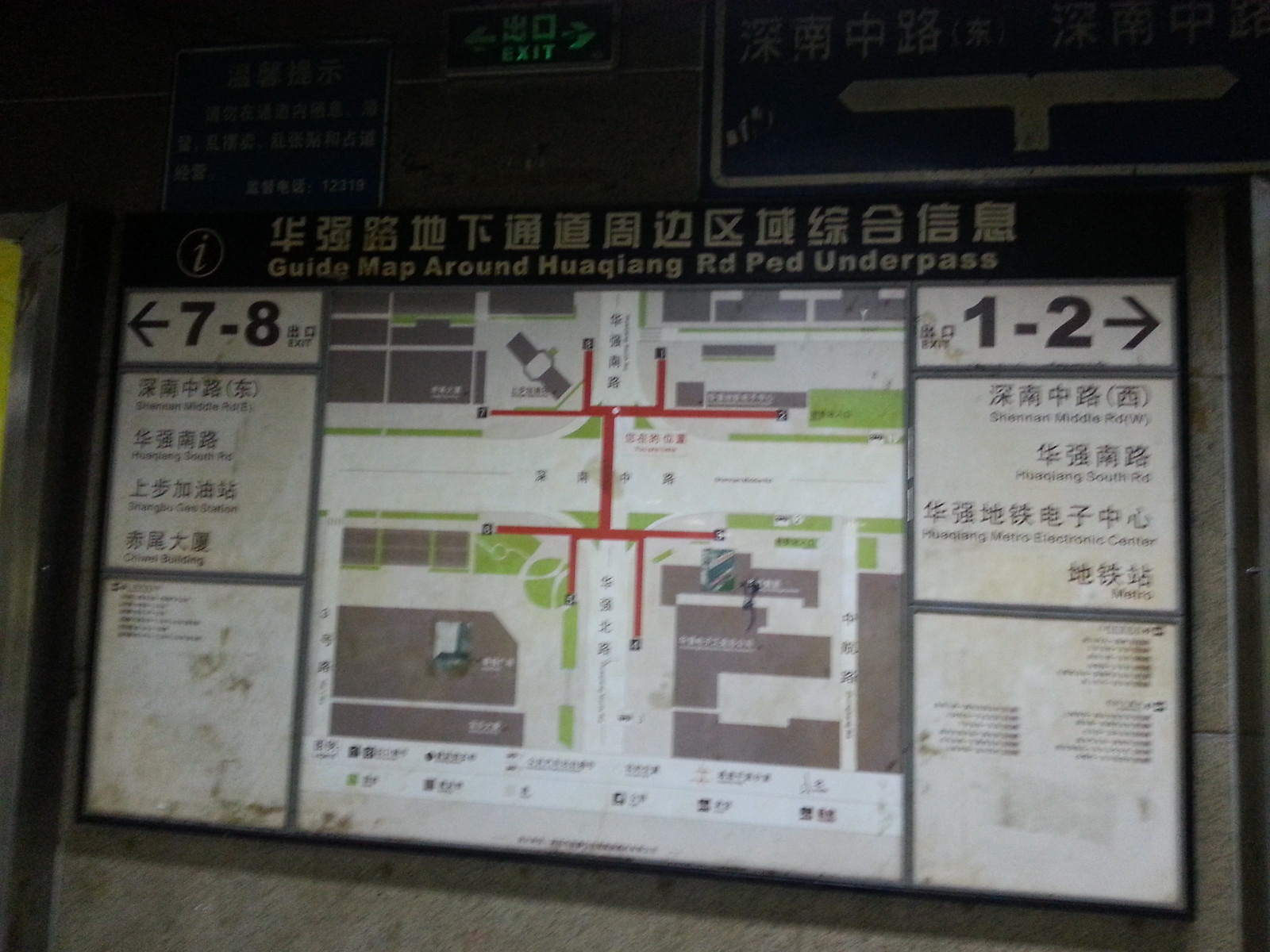The photograph showcases a large, framed rectangular map titled "Guide Map Around Huaqing Road Pedestrian Underpass" in white text set within a black rectangle at the top center. Directly above this title are Chinese characters. The map itself, positioned prominently in the center, displays detailed diagrams of streets, buildings (depicted in gray), and grassy areas (marked in green). Flanking the map, clear directional indicators are seen: on the left, "7 to 8" with an arrow pointing left, and on the right, "1 to 2" with an arrow pointing right, each accompanied by corresponding Chinese characters and English labels explaining various locations. The map is mounted on a stone grey wall, and is accentuated by multiple signs above it: blue signs with white Chinese characters, and a conspicuous black and green EXIT sign, illuminated with light.